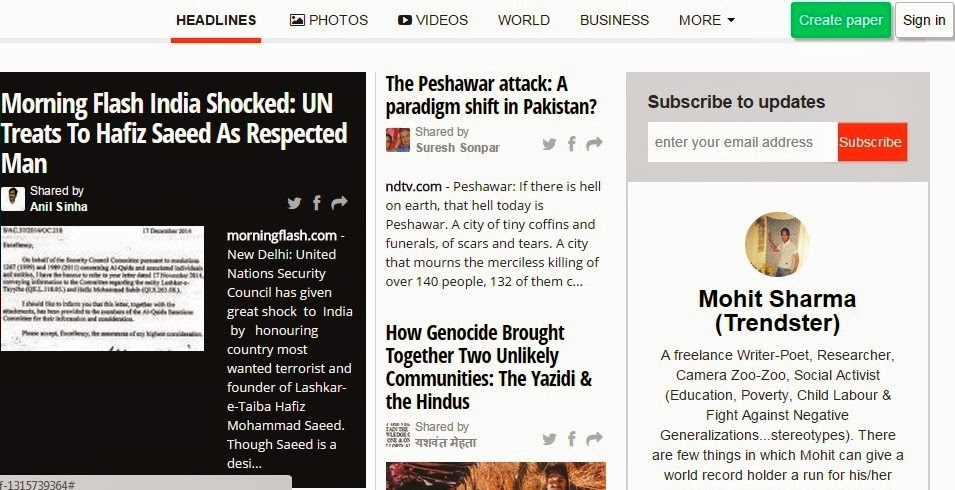This is a screenshot of a news webpage featuring a comprehensive layout with various sections. At the very top, there's a white menu bar with options labeled "Headlines," "Photos," "Videos," "World," "Business," and a "More" dropdown menu. In the upper right-hand corner, a green button labeled "Create Paper" is positioned beside a white "Sign In" button. 

Beneath this menu bar lies the main content area. On the left-hand side, there is a rectangular segment with a black background and white text displaying "Morning Flash," an urgent news alert. The headline reads, "India Shocked, UN Treats Hafiz Saeed as Respected Man." 

At the center of the page, there is a narrow white column featuring two news articles: the first one is titled "The Peshawar Attack," while the second is "How Genocide Brought Together Two Unlikely Communities: The Yazidi and the Hindus."

On the right-hand side, there is a user profile section with a profile picture and the name "Mohit Sharma," who is identified as a "Trendster." Above his picture is an invitation to "Subscribe to Updates" with a field to enter an email address. Below Mohit Sharma’s name, a brief bio is provided.